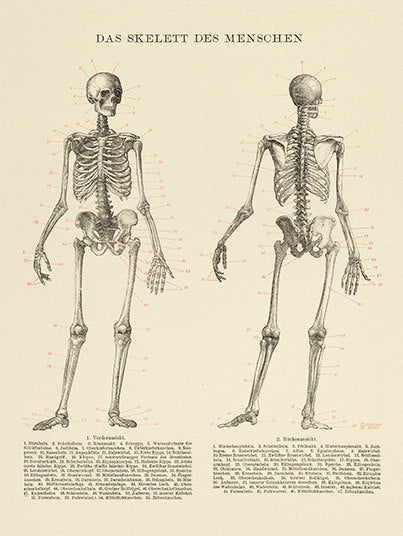This image is a detailed photograph of a page from a German book, likely a medical text, illustrating the various parts of the human skeleton. At the top of the page, in bold black text, the title reads "Das Skelett des Menschen" (spelled D-A-S space S-K-E-L-E-T-T space D-E-S space M-E-N-S-C-H-E-N). The page features two detailed drawings of the human skeleton: the left drawing presents an anterior view while the right drawing provides a posterior view. Both skeletons are intricately labeled with red numbers and corresponding red lines pointing to every bone. The numbers likely relate to an index or legend, which appears as two columns of text at the bottom of the page. However, this text is blurry and too low resolution to read clearly. The overall design is rendered on a light brown background with black lines for the skeletons and text, emphasizing the anatomical details with a classic, educational style.